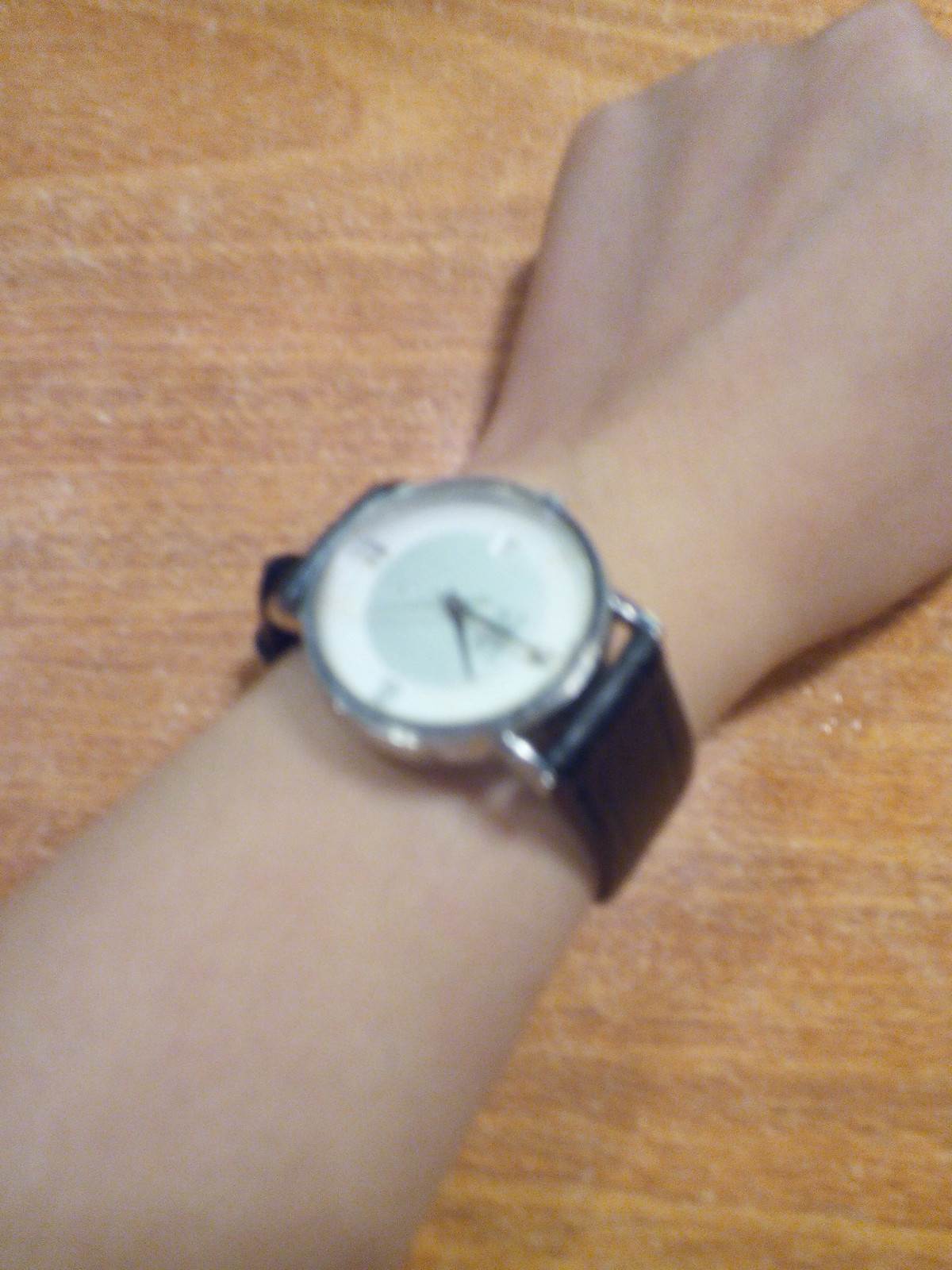A detailed photograph captures a wooden tabletop as the background. Resting on the surface is a green object, although its exact nature is unclear. In the foreground, a person’s arm extends into the frame, with visible veins and a pronounced knuckle on the hand. The wrist is adorned with a silver-bodied watch, featuring a glass face. The minute hand of the watch points to the 6 o'clock position, while the hour hand lies between the 6 and 9 o'clock marks. The watch is secured with black leather wrist straps, adding a touch of sophistication to the overall scene.